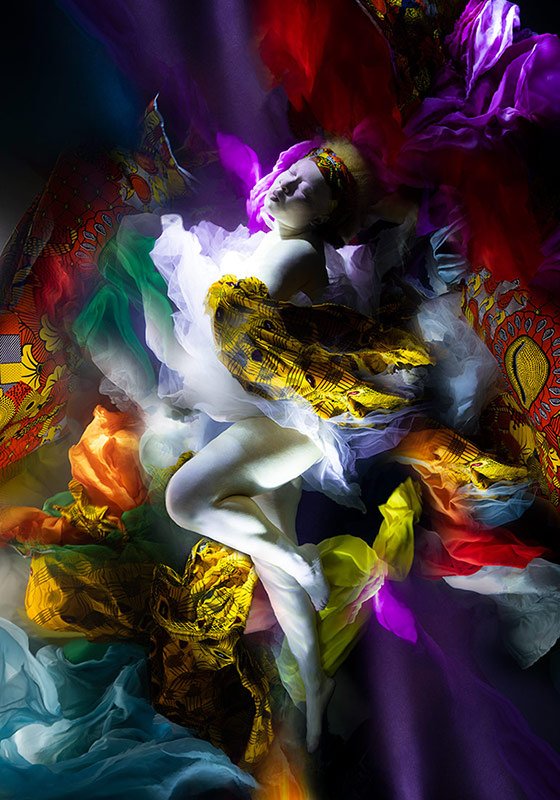The image is a vibrant and dreamlike portrayal of an albino woman with a very pale, almost unnatural white complexion, and short blonde hair adorned with a colorful headband. She is the central figure in a collaborative piece of art and photography, lying on a myriad of colorful fabrics that cascade around her. Her body is positioned in an S-line with one leg bent and the other straight. Her eyes are closed and her head is tilted back, illuminated by a white light that casts a serene glow on her face. She is semi-naked, with her intimate areas modestly covered by a prominent yellow patterned fabric reminiscent of tartan, and ethereal pieces of white twill or silk. Surrounding her are rich arrays of purple, red, yellow, blue, orange, and green fabrics, creating an artistically textured and colorful scene.